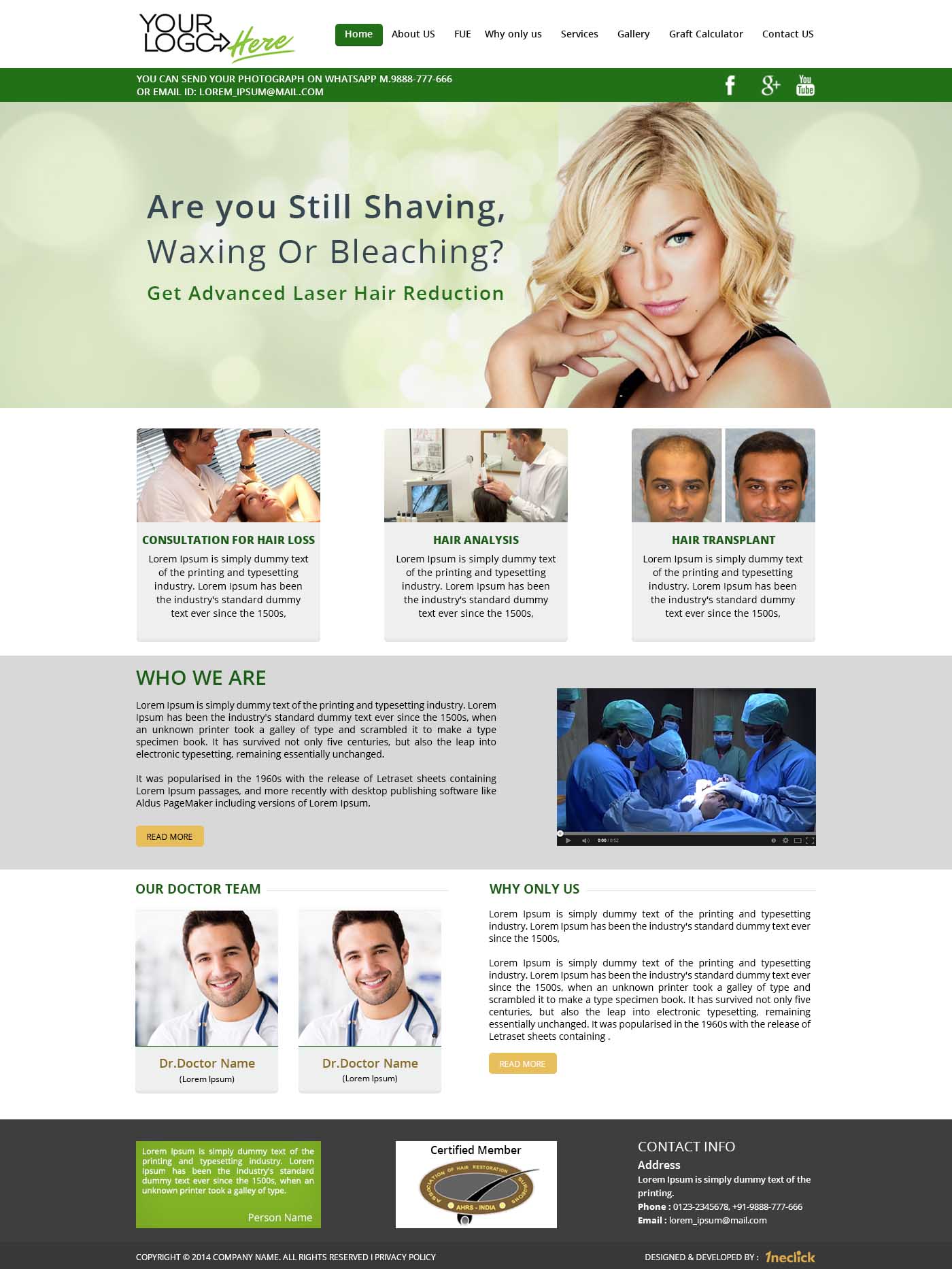This image depicts a promotional page featuring multiple segments of information and visual content. At the top of the page, there is a placeholder marked "Your Logo," accompanied by an arrow pointing to the text "here." Below this section, instructions are provided, stating that photographs or other content can be sent via WhatsApp, with a series of placeholder numbers listed for contact. An email option is also given, using a placeholder address: lorem_ipsum@mail.com.

The next section contains a promotional message addressing individuals who are still using traditional hair removal methods like shaving, waxing, or bleaching. It suggests opting for advanced laser hair reduction. This section is enhanced with the image of a blonde woman with wavy hair, dressed in a black tank top, gazing contemplatively out from beneath her bangs.

Underneath this promotional message are three boxes, each representing different services. The first box shows an image of a professional, possibly a dermatologist, consulting with a patient, and is captioned "Consultation for Hair Loss." All the text within these boxes is placeholder text (Lorem ipsum), commonly used in the printing and typesetting industry:

1. **Consultation for Hair Loss:** 
    - Caption: Lorem ipsum is simply dummy text of the printing and typesetting industry. Lorem ipsum has been the industry's standard dummy text ever since the 1500s.

2. **Hair Analysis:** 
    - Caption: Lorem ipsum is simply dummy text of the printing and typesetting industry. Lorem ipsum has been the industry's standard dummy text ever since the 1500s.
    
3. **Hair Transplant:** 
    - Caption: Lorem ipsum is simply dummy text of the printing and typesetting industry. Lorem ipsum has been the industry's standard dummy text ever since the 1500s.

The repetition of placeholder text suggests that this is a draft or template for the final promotional material.